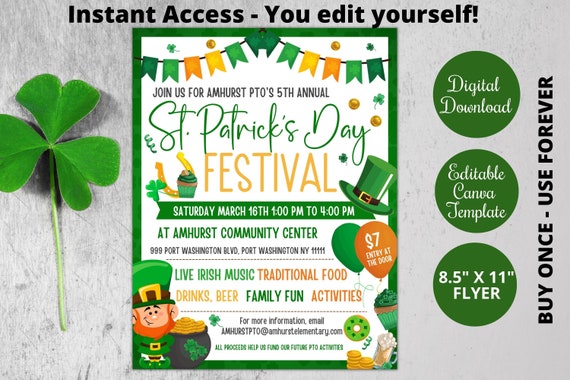The image showcases an editable Canva template for a flyer, providing instant access for personalized edits. At the top, it features bold black text stating "Instant Access, You Edit Yourself," and on the vertical right side, it advertises "Buy Once, Use Forever." The template itself is an 8.5 by 11-inch digital download, highlighted in three green circles to the right, with the text "Digital Download," "Editable Canva Template," and "8.5x11 Flyer."

The sample flyer within the template promotes the Amherst PTO's 5th Annual St. Patrick's Day Festival. It features a green-bordered design with a colorful banner of ten flags in shades of green, light green, orange, and yellow. At the top, black text reads "Join us for Amherst PTO's fifth annual," followed by green text declaring "St. Patrick's Day" and black text saying "Festival." Essential details are neatly displayed: Saturday, March 16, from 1 p.m. to 4 p.m. at the Amherst Community Center, located at 999 Port Washington Boulevard, Port Washington, New York, 11050. The event promises live Irish music, traditional food, drinks, beer, and family fun activities, for an entry fee of $7 at the door, highlighted inside an orange balloon at the bottom right.

Additional visual elements include a leprechaun with a pot of gold on the bottom left, festive green items on the bottom right, and a three-leaf clover on the left side of the image. For inquiries, an email is provided: AmherstSTEP2@amherselementary.com. All proceeds support future PTO activities.